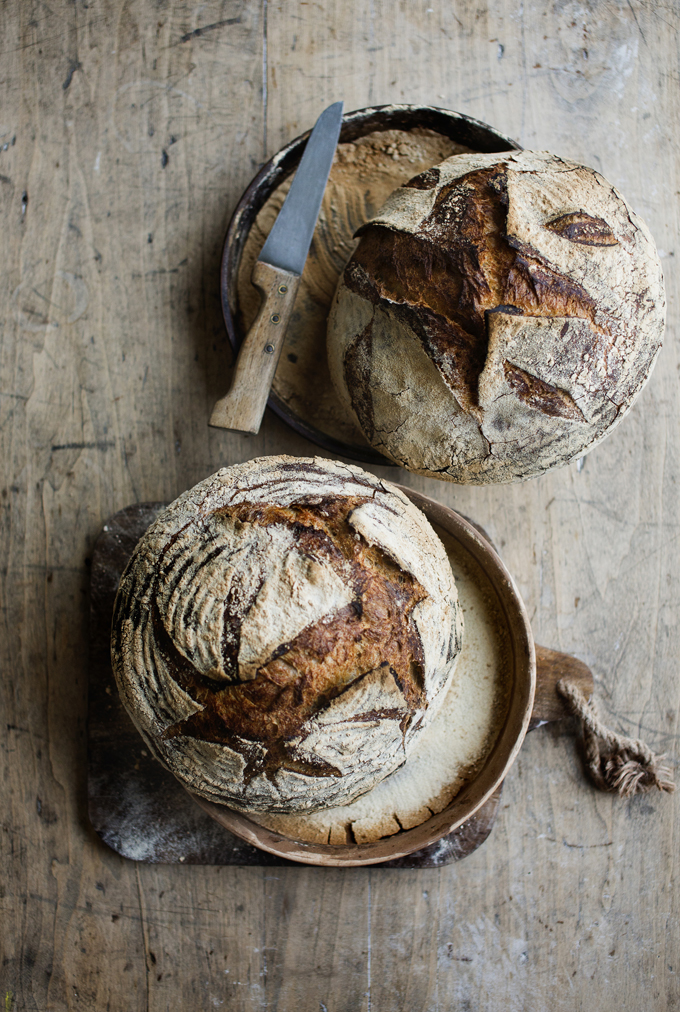This image showcases two freshly baked, rustic round loaves of bread, presented with an inviting, well-lit, and homey appeal. Both loaves rest on a well-used, light wooden table marked with various cut lines, adding to the scene's rustic charm. The larger loaf, adorned with intricate, flour-dusted patterns on its dark golden crust, reclines on a plate that sits atop a wooden cutting board with a handle and a rope attached. The second loaf rests on a stone plate, tilted slightly downward, enhancing the natural elegance of the presentation. A knife with a wooden handle, positioned beside the top loaf, suggests readiness for slicing. The entire tableau, with its seamless blend of browns and tans from the table, cutting board, and bread, creates a warm and earthy atmosphere.